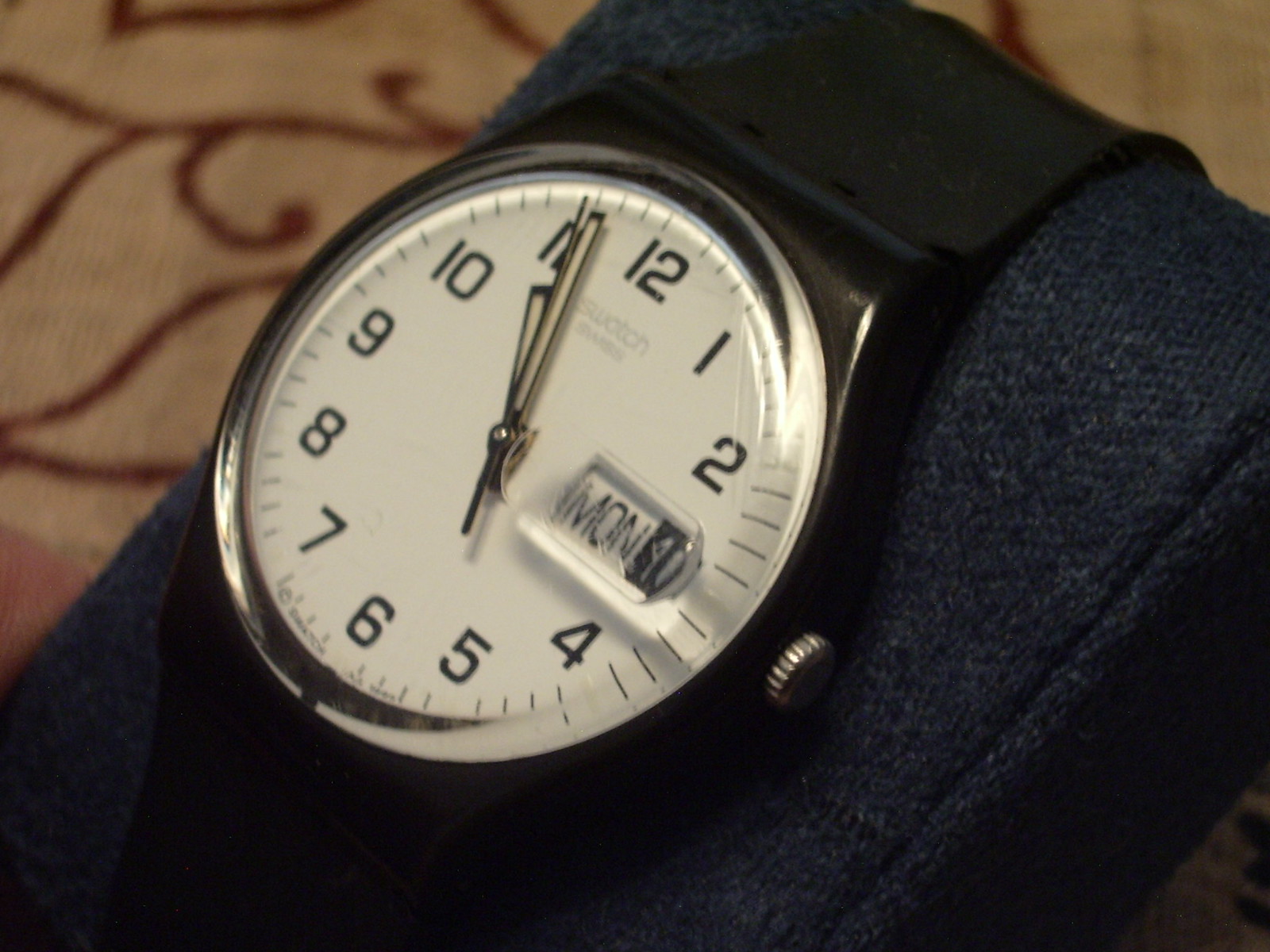This is a detailed close-up image of a wristwatch meticulously displayed. The watch is set against a dark blue background, resembling the case in which it might be packaged when purchased. The watch itself features a white face with bold black numerals from 1 to 12 and a window indicating the day, which reads "M-O-N" for Monday. The date also appears beside the day but is displayed differently, as accounts vary between a number 1 and a number 4. The time on the watch reads approximately 10:56 or a few minutes before 11 o'clock. The watch has a black band, complemented by a silver winding dial on its side. Behind the watch is a backdrop of tan-colored material patterned with organic, maroon squiggly lines. The hands, including the hour, minute, and second, are distinctly visible, adding to the clarity and functionality of this elegant timepiece.